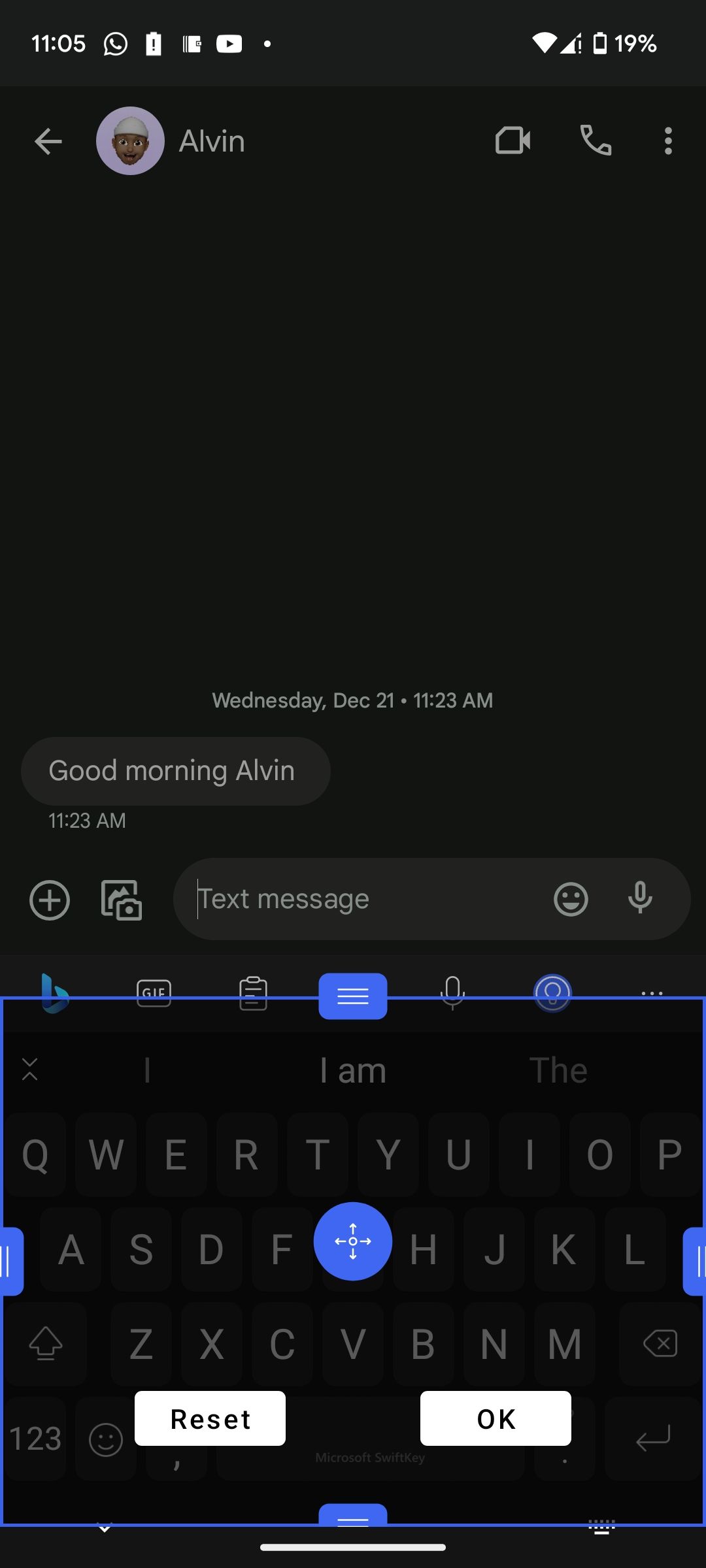A detailed descriptive caption for the image could be:

"Portrait-oriented screenshot taken from a smartphone, showcasing a messaging app interface. At the top left corner, the screen displays the time as 11:05, accompanied by a dialogue icon, battery indicator, and two unrecognized icons. On the right side, icons show Wi-Fi strength, cellular signal, and a battery level at 19%. Below, a white circular icon with a face and the name 'Alvin' appears. To the right of this, icons for the camera, phone, and three vertical dots are present. Near the bottom, a message timestamped Wednesday, December 21st, 11:23 AM reads, 'Good morning, Alvin.' An open text message box with a visible keyboard is prepared for a reply. The interface features a black background with predominantly white text. Surrounding the keyboard is a blue outline that includes options labeled 'OK' and 'Reset.'"